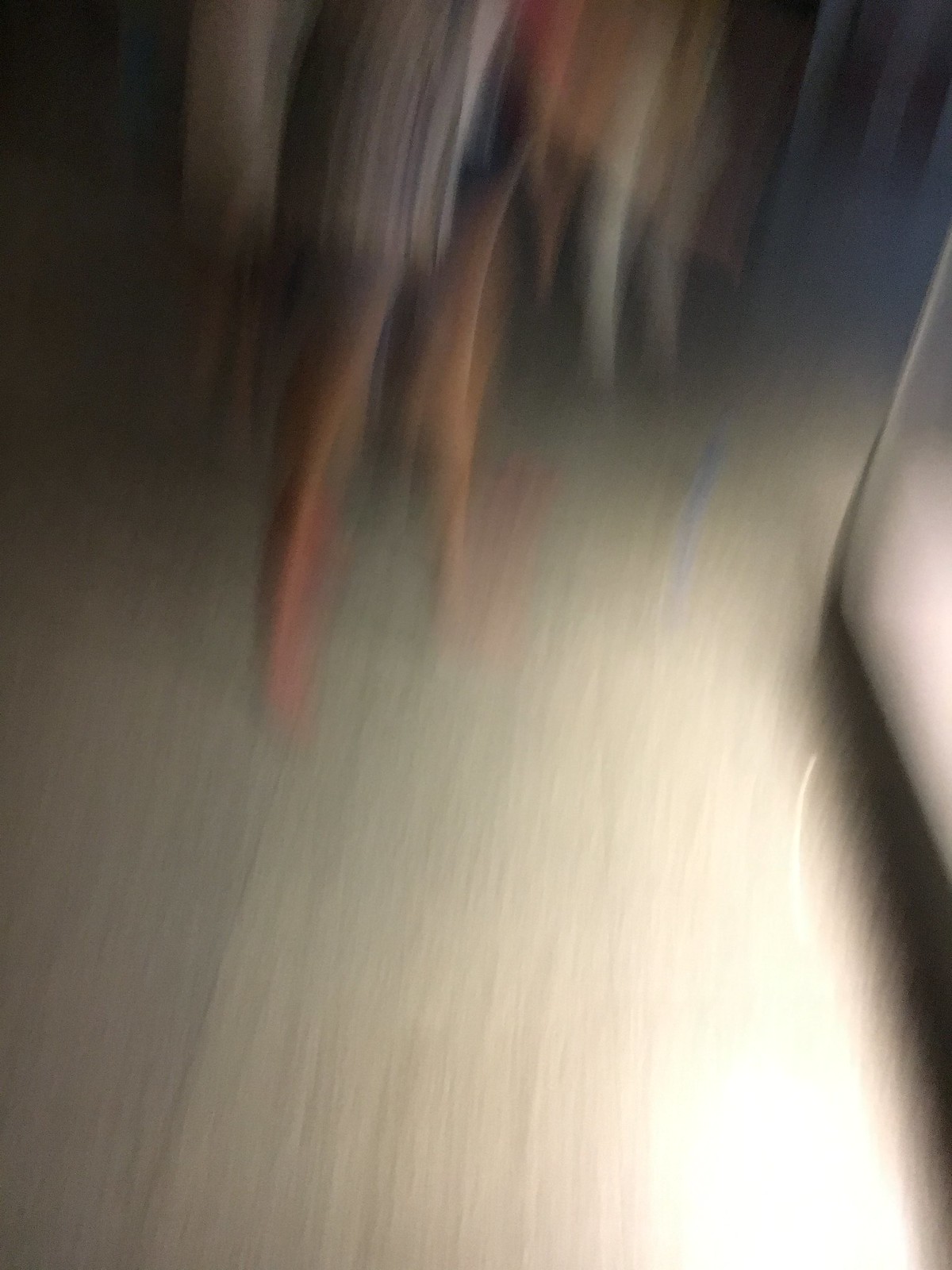This image captures a dynamic blur, conveying a sense of movement. The entire scene is a cascade of colors, primarily devoid of sharpness, creating a feeling of continuous motion. At the bottom of the image, there seems to be a flooring with hues reminiscent of bamboo, painted in shades of yellow and light brown. The lower right corner is particularly bright, washed out by intense lighting. Above this, a distinct black line emerges at an angle, forming a sort of triangular shape. This line adds to the movement, as if an object is darting through the image. The background features a vivid display of brushstroke-like lines descending vertically. These strokes are predominantly orange, interspersed with sections of purple, off-white, orange again, and green. Collectively, the colors and brushstroke textures lend an abstract, painterly effect, suggesting a blend of artistic motion and vibrant energy.